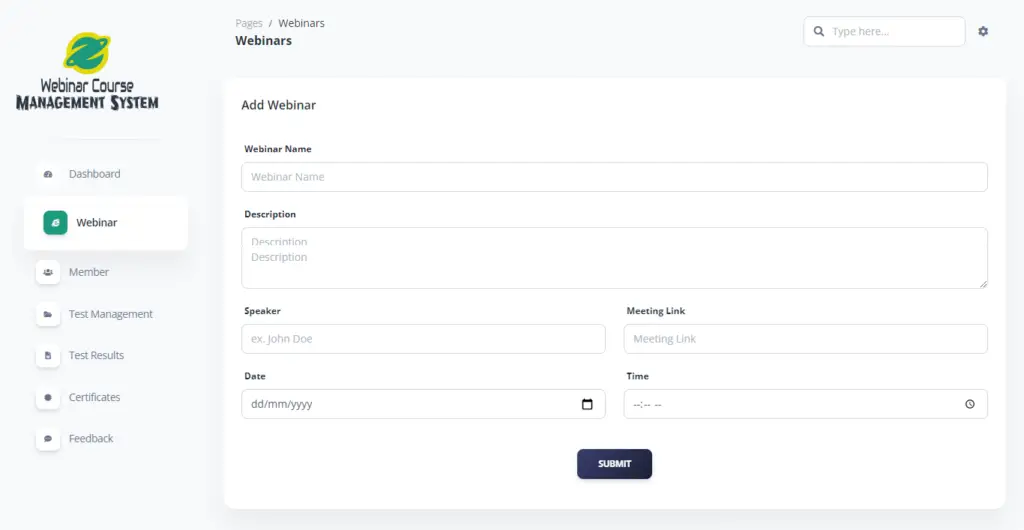The image showcases a detailed layout of a webpage dedicated to managing webinars. At the very top of the page, the breadcrumb navigation reads "Pages / Webinars" with the "Webinars" section highlighted in black text. Below this, there is a prominent "Add Webinar" heading, under which several fields are presented for user input.

The fields include: 
1. **Webinar Name:** A blank text box awaiting user input.
2. **Description:** A larger text box for entering a detailed description of the webinar.
3. **Speaker:** An example entry, "John Doe," is displayed, indicating where the speaker's name should be entered.
4. **Meeting Link:** A text box for inputting the URL of the webinar meeting.
5. **Date and Time:** A section for specifying the date and time of the webinar.

At the bottom of this section, there's a "Submit" button to finalize the entry.

On the left side of the page, there is a sidebar labeled "Webinar Course Management System," featuring a green and yellow circular icon. This sidebar contains several navigation tabs, each accompanied by its respective icon. The tabs listed are:
- Dashboard
- Webinar
- Member (icon depicting multiple people)
- Test Management
- Test Result (file icon)
- Certificates (represented by a gray circle icon)
- Feedback (chat message icon)

The sidebar text is in gray and does not dominate the screen space. Instead, the primary focus of the page is the "Add Webinar" section with its various input fields.